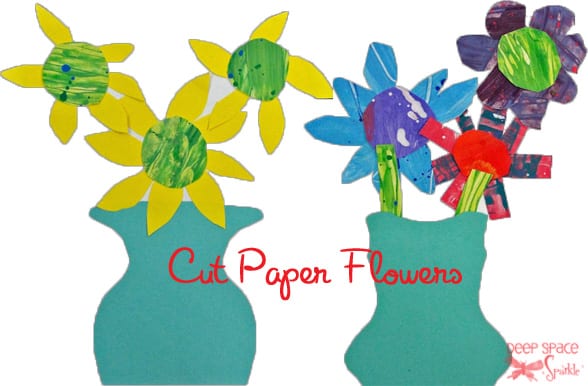The image titled "Cut Paper Flowers" showcases a computerized artwork featuring two intricately designed vases with flowers, crafted to appear as if made from paper. Centered in the image is the title written in red text. On the left side, the green vase has a distinctive shape with a wide opening, narrowing to a metal-like neck before widening again to a flat base. This vase contains flowers resembling bright green centers with mustard yellow petals, akin to daisies or sunflowers. On the right, another green vase has a unique form reminiscent of the top of a woman's sleeveless shirt, curving inwards and then outwards. This vase holds a variety of colorful flowers: a blue flower, a red flower, a purple flower with a green center, and a flower with purple petals and a green center. Both vases exhibit a mix of vibrant colors and creative designs, blending elements of nature with artistic expression. The detailed portrayal of each flower and vase emphasizes the artwork's intricate and imaginative approach to floral design.